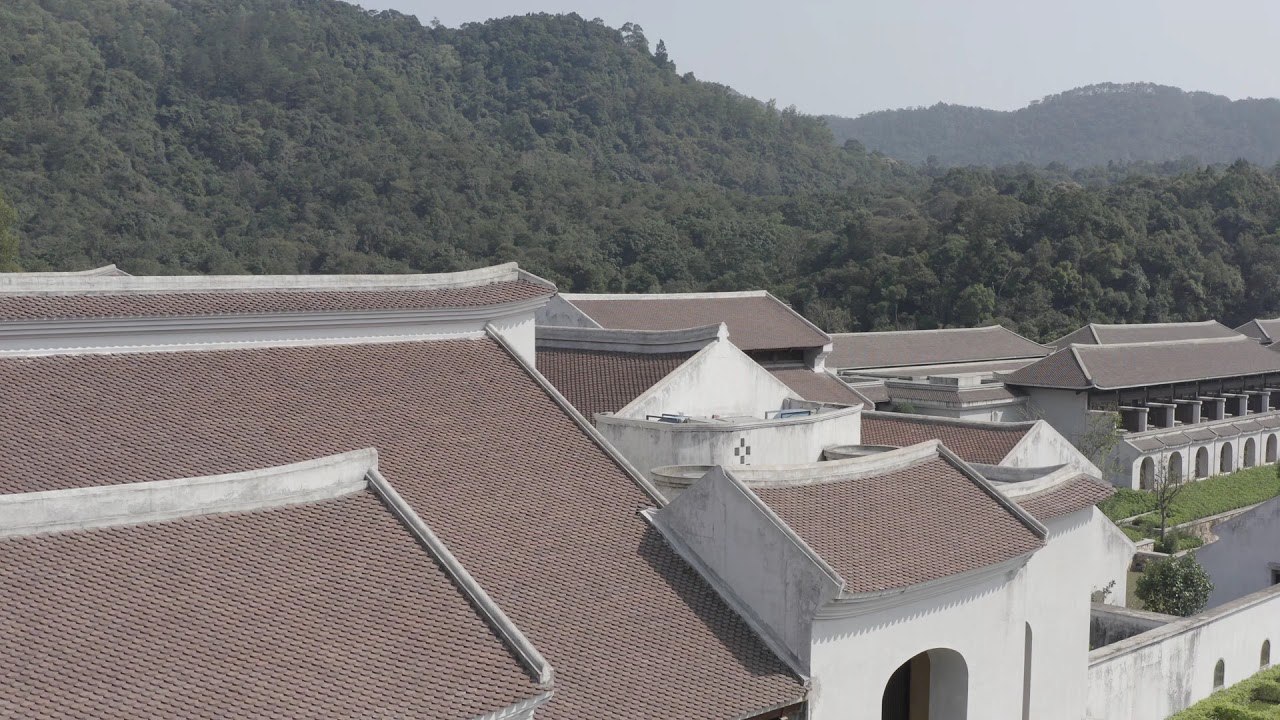The photograph depicts a cluster of buildings nestled in a hilly, forested area. The buildings, constructed from a mix of white and gray stone, feature a variety of arched entryways and windows. Their tiled roofs, a dark orange-amber color, are predominantly sloped in different directions. Some buildings are supported by columns on the far right side, creating a series of arches beneath the concrete walls. The structures, possibly inspired by East Indian or Asian architectural styles, stand two to three stories tall and are tightly packed together. Surrounding the buildings are patches of grass, trees, and bushes, enhancing the secluded, serene atmosphere. In the background, densely forested mountains rise prominently, their thick greenery completely obscuring the ground. The distant hills appear slightly hazy under a gray sky, adding to the tranquil, remote setting.